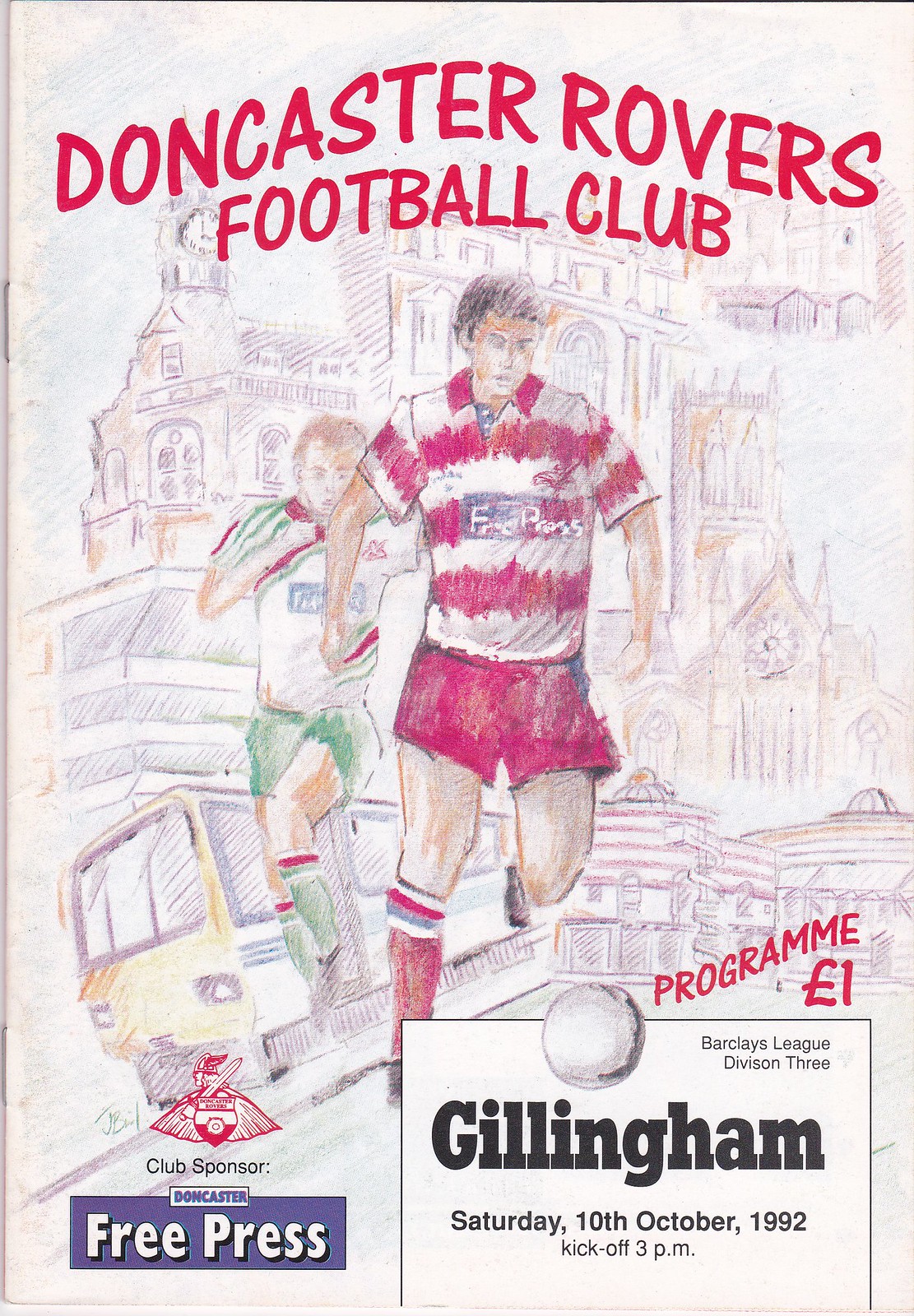The image portrays the cover of a soccer program for a match between Doncaster Rovers Football Club and Gillingham, which took place on Saturday, 10th October 1992, with a kickoff at 3 p.m. The cover is a vertical, rectangular sketch in colored pencils, framing an action-packed scene of two soccer players. The player in the foreground, donning a red and white uniform, is running towards the viewer, dribbling a soccer ball, while a second player in a green and white uniform with blondish hair chases him from behind. Both players are detailed with red and green shorts, respectively, and the appropriate matching socks and shoes.

The background diverges from the soccer field, instead depicting a series of pale-colored sketches of buildings, including a clock tower, a church, and houses, suggestive of a cityscape, possibly London. Among these city elements, a bus and a train can be seen, rendered in muted yellows, blues, browns, and occasional purple tones, creating a dynamic backdrop.

Text on the cover includes key details such as "Doncaster Rovers Football Club" at the top, along with "Program, Barclays League Division III, Gillingham, European One." Notably, the term "PROGRAMME" appears in the lower right, suggesting a potential linguistic nod (perhaps Spanish). The artwork is further credited to sponsors and advertisements, like the "Doncaster Free Press," showcasing a strong dedication and community connection through its original and vivid artistic style.